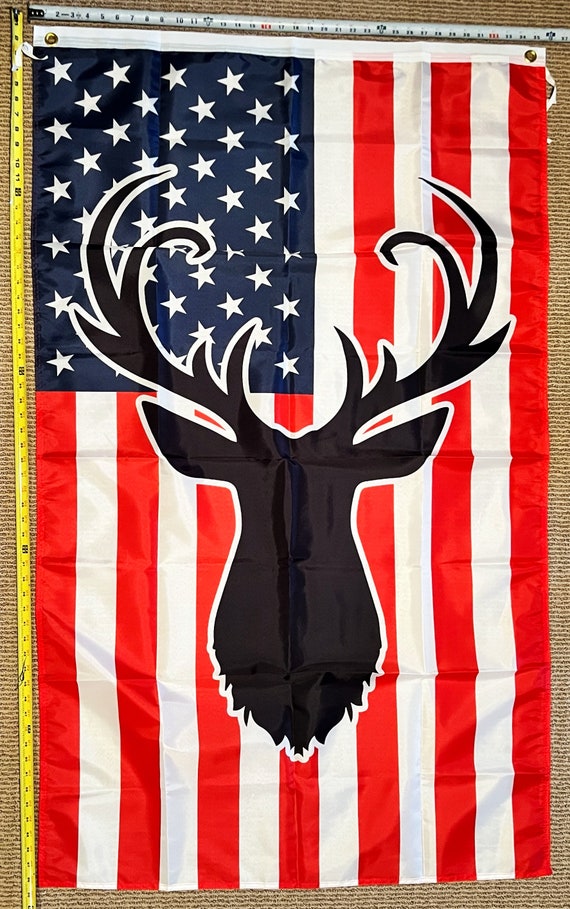The photograph captures a large American flag, characterized by its familiar navy blue square adorned with white stars and its alternating seven red and six white stripes. At the center of the flag, a striking black silhouette of a deer head with antlers is situated, bordered by a thin white outline. The flag shows signs of having been previously folded, evident from the noticeable creases running across its fabric. The backdrop is a cardboard surface etched with numerous lines and hatches. Along the left side of the flag runs a yellow measuring tape, stretching vertically, while a light blue measuring tape spans horizontally across the top. Additionally, at each corner at the top of the flag, there are eyelets. A concealed item peeks out from beneath the top right of the flag.